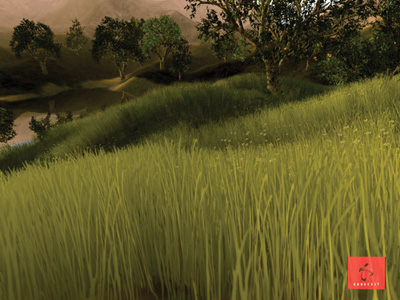This digital illustration depicts a serene landscape characterized by gentle hills covered in long, tall grass that undulate across the bottom portion of the image. In the background, a series of hills and trees curve gracefully from the top right to the center left, creating a dynamic diagonal composition. At the left center, there is a tranquil body of water, perhaps a lake, reflecting the surrounding scenery. The colors of the image are reminiscent of a Renaissance painting, lending it a timeless and classical aesthetic. The sky above is a dramatic mix of cloudy reddish-gray tones, adding depth and mood to the scene. Highlights on the tall grass in the foreground and mid-ground enhance the texture and realism of the vegetation. At the bottom right corner, there is a square red logo featuring an intricate design, suggesting the image may be intended for use in web design or digital media applications.